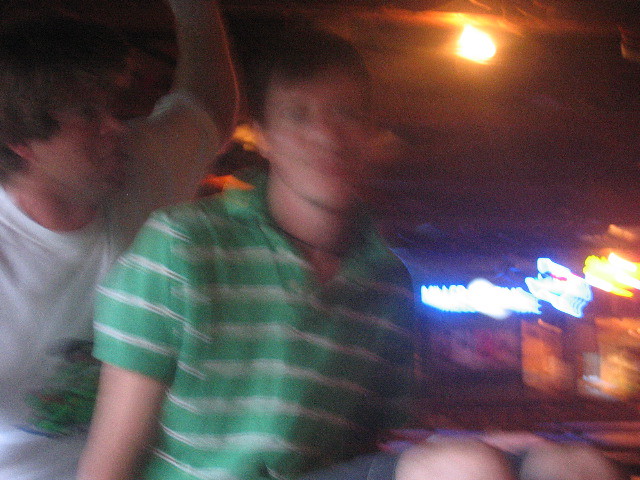An out-of-focus image features a dark, gloomy sky with the Sun faintly visible in the top right-hand corner. In the foreground, two people are seated. The person on the left has dark hair and is wearing a white shirt adorned with a green pattern on the front. The individual on the right also has short, dark hair and is dressed in a green and white striped, short-sleeved t-shirt. At the bottom of the image, there are two pinkish areas, likely indicating the person's knees, with a hint of gray shorts visible. Street lights are seen in the blurry background, adding to the dim ambiance of the scene.